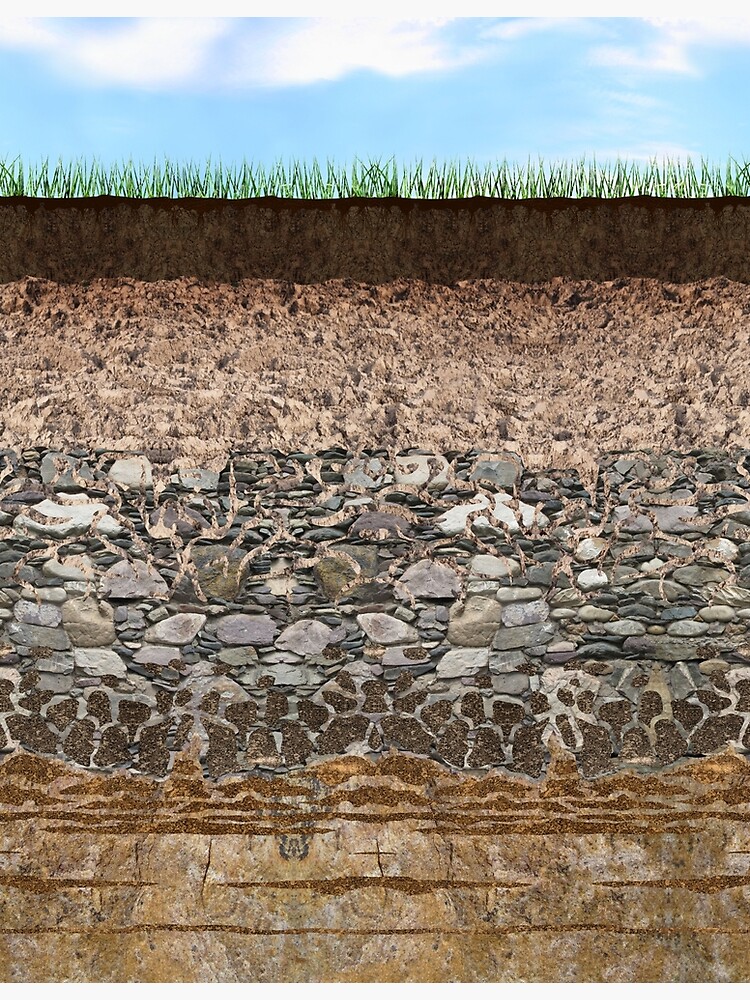This scientific image is a detailed cross-section of soil and the underlying geological strata, depicting various layers from the surface to the bedrock. At the very top, the image features a serene light blue sky with wispy white clouds. Just below this, there is a layer of short, sprawling grass. Immediately beneath the grass, a dark brown topsoil layer is visible, approximately an inch thick. This is followed by a slightly lighter band of soil or clay, twice as thick as the topsoil, which appears more compact and rocky. Below this, a considerable layer of sedimentary material emerges, displaying a pattern of large rock chunks interwoven with sparse soil. This sedimentary layer transitions into an even deeper, thicker band that resembles the prior rocky layer but is marked by larger, distinct rock formations. Finally, at the bottom, a solid bedrock layer emerges, characterized by its reddish, porous, and unyielding nature, indicating it has remained unchanged for millions of years. This cross-section visually encapsulates the gradual formation and variation of soil and rock layers over geological time, providing insights into the complex buildup of the earth's crust that supports plant life on the surface.